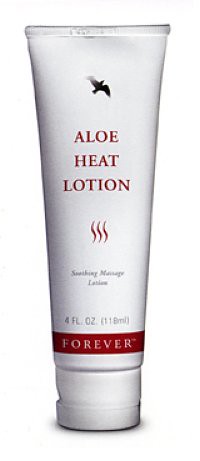The image features a pristine, four-ounce white tube of Aloe Heat Lotion standing upright on a white table. The cap is white, flip-top, and casts a noticeable shadow on the table. The tube is adorned with a detailed graphic of a black bird in flight near the top. Directly below the bird, the name "Aloe Heat Lotion" is prominently displayed in a reddish-pink font. Underneath this title, three vertical, wavy lines appear in the same reddish-pink color, symbolizing rising heat. Further down, the text "Soothing Massage Lotion" is inscribed in a small, dark script. The tube also specifies "4 fl. oz. (118 ml)" in black letters. At the very bottom, a reddish-pink band encircles the tube, with the word "FOREVER" written in bold block white letters, and a small "TM" symbol next to it. The clean, minimalist background and the straightforward, head-on photo composition suggest that this image is likely intended for an advertisement, showcasing the product in new and unused condition.